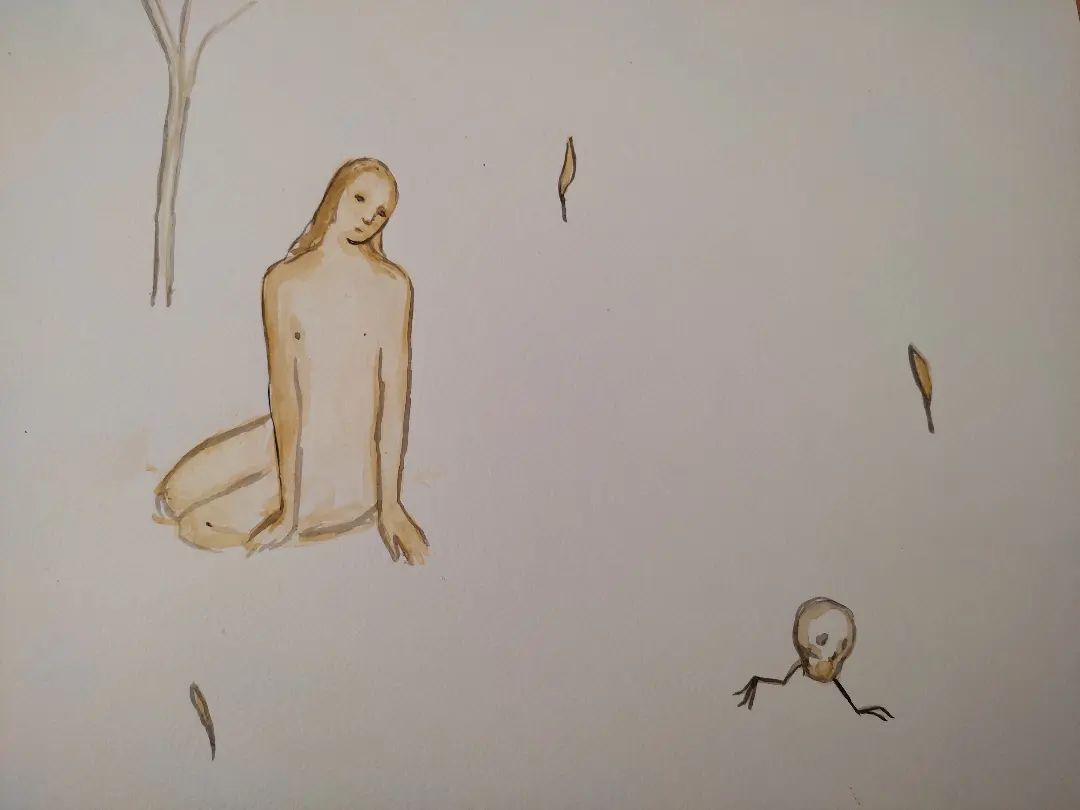The drawing features a stark white background, with most of the surface left as blank space. In the upper left portion of the image, there's a thin, bare tree with two prominent branches and a third branch emerging towards the top, although the top part of the tree is cut off in the frame. Positioned centrally below the tree is a nude woman, depicted with minimal detail. She has long hair that partially covers her face and cascades past her shoulders. She is seated with her knees tucked beneath her, her palms placed in front of her on the ground, and she appears to be gazing longingly towards the lower right corner. In this corner, there's an intriguing small skull with slender black bird legs, giving the impression of movement as it seems to be walking away from the woman. Scattered throughout the image are three small, abstract brown leaves: one in the upper portion, one in the lower left corner, and one on the right side.